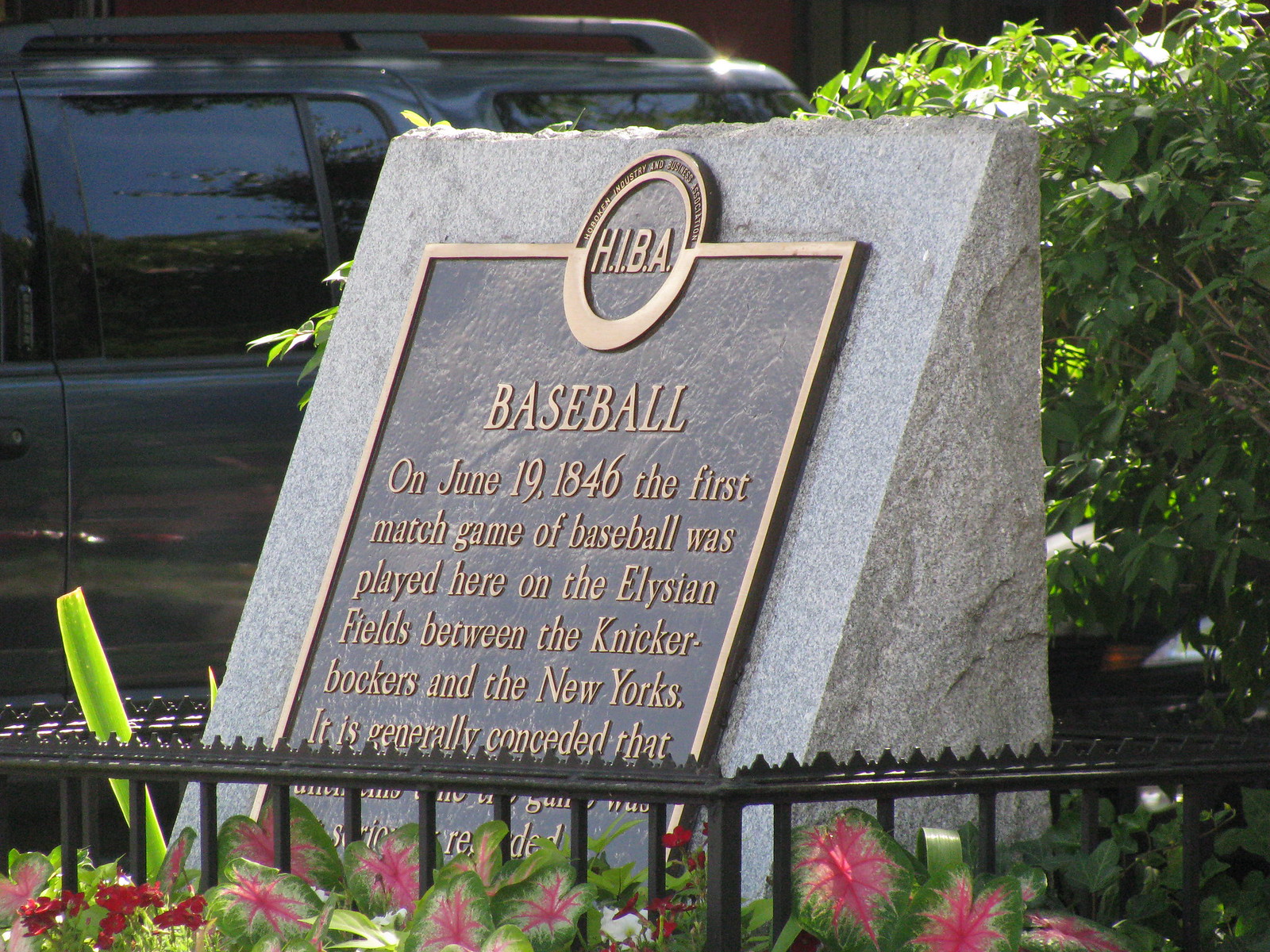The horizontal rectangular image captures a historically significant granite plaque, resembling a tombstone, in a park setting. This memorial is enclosed by a black metal fence and surrounded by vibrant, well-tended flowers, including purple, green, and red blossoms. In the background, on the right, a lush green bush can be seen, while on the left, there are parked vehicles, including a dark-colored SUV with tinted windows, indicating proximity to a parking area.

The plaque at the center of the granite stone prominently features the initials "H-I-B-A" encircled by brass. Below, in large letters, it reads "Baseball." The inscription commemorates the first match game of baseball, which took place on June 19, 1846, on the Elysian Fields between the Knickerbockers and the New Yorks. Due to the angle of the fence, some of the text is obscured, but it is clear that the plaque captures an essential moment in baseball history.